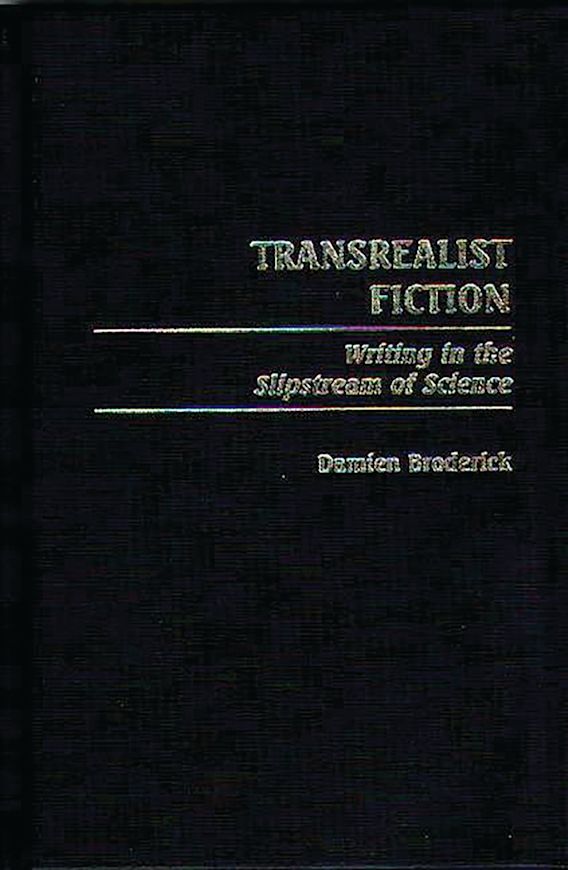This is a rectangular image, approximately six inches high and three inches wide, featuring the front cover of a book. The cover has a black background with a woven fabric texture, visibly showing crisscross lines. About a third of the way down, slightly to the right of center, the title "Trans Realist Fiction" is prominently displayed in large, bold print across two lines. Beneath the title, a thin, horizontal bar spans left to right with a blur of whitish-yellow and hints of color such as purple. Below this bar, the subtitle "Writing in the Slipstream of Science" is printed, followed by another thin, similarly colored bar. At the bottom of the cover, the author's name, "Damian Broderick," is written in the same whitish-yellow, blurred style. The image overall is somewhat blurry, indicating it might not be a high-quality photo.